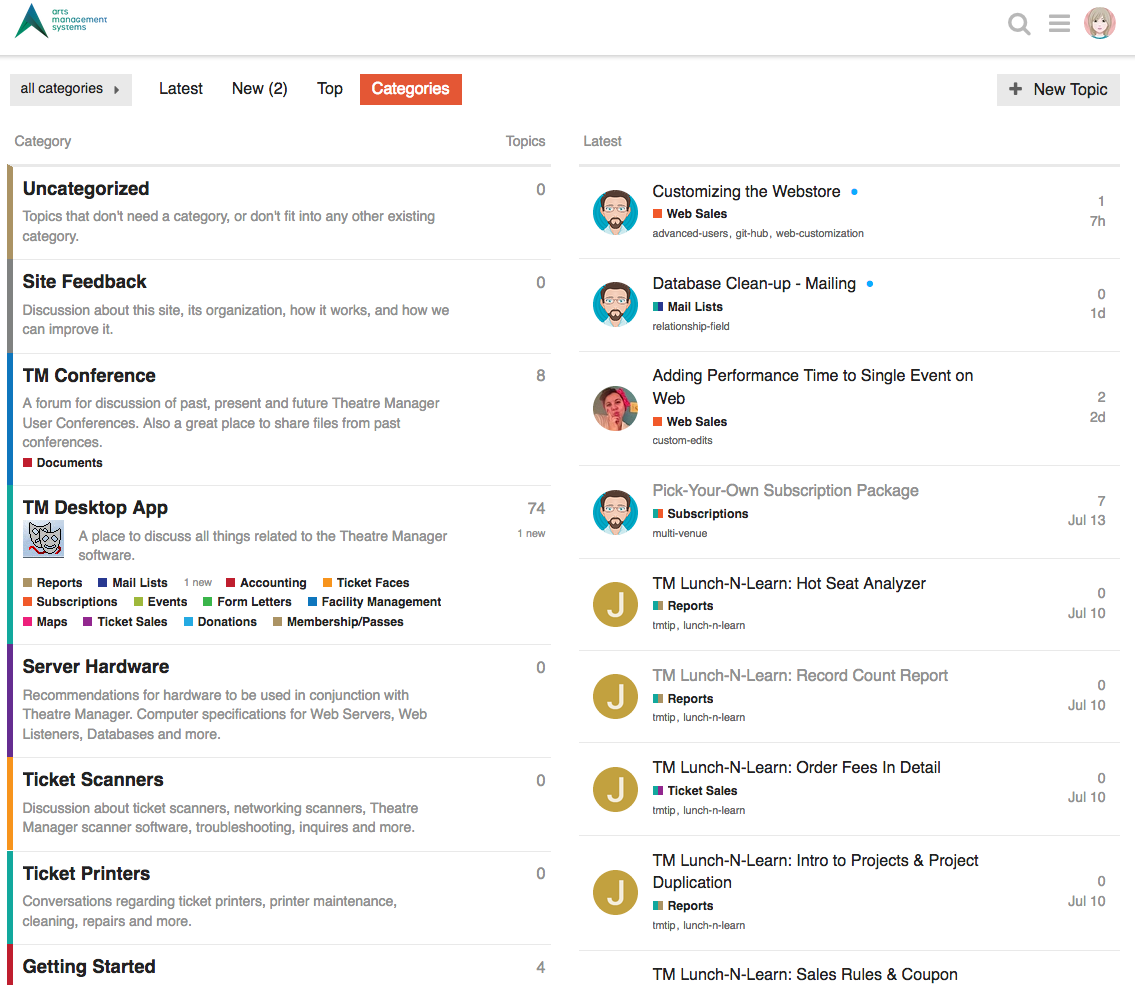Screenshot of a website titled "Arts Management Systems" with a navigational menu at the top, displaying options: All Categories, Latest, New to Top, and Categories. The "Categories" section is selected by default.

In the "Category" section, several sub-sections are listed:

1. **Uncategorized**
   - Description: Topics that don't need a specific category or don't fit into any existing category.
   - Topics: 0

2. **Site Feedback**
   - Description: Discussions about the website's organization, functionality, and potential improvements.
   - Topics: 0

3. **TM Conference**
   - Description: Forum for discussing past, present, and future Theater Manager user conferences, and sharing files from previous conferences.
   - Topics: 8

4. **Documents**
   - Description: Repository for various files and documents.

5. **TM Desktop App**
   - Description: Platform to discuss anything related to Theater Manager software, covering areas such as reports, mail lists, accounting, ticket faces, subscriptions, events, form letters, facility management, maps, ticket sales, donations, memberships, and passes.
   - Topics: 74 (1 new)

6. **Server Hardware**
   - Description: Recommendations for hardware to be used with Theater Manager, including computer specifications for web servers, web listeners, databases, etc.
   - Topics: 0

7. **Ticket Scanners**
   - Description: Discussions about ticket scanners, networked scanners, Theater Manager scanner software, troubleshooting, and inquiries.
   - Topics: 0

8. **Ticket Printers**
   - Description: Conversations regarding ticket printers, including maintenance, cleaning, repairs, and more.
   - Topics: 0

9. **Getting Started**
   - Topics: 4

On the right side of the page, topics related to "Customizing the Web Store" and advanced Theatre Manager features are displayed:

- Customizing the web stores: Web sales, advanced users, GitHub, web customization, and database cleanup.
- Mailing: Mail lists, relationship field, adding performance time to single events on the web, and custom edits.
- Subscription packages: Pick your own, multi-venue.
- TM Lunch and Learn series covering various topics:
  - Hot Seat Analyzer
  - Record Count Report
  - Order Fees in Detail
  - Intro to Projects and Project Duplication
  - Sales Rules and Coupons

Each "TM Lunch and Learn" session is tagged as reports, tips, ticket sales, and related fields, demonstrating a focus on thorough professional development within the system’s user community.